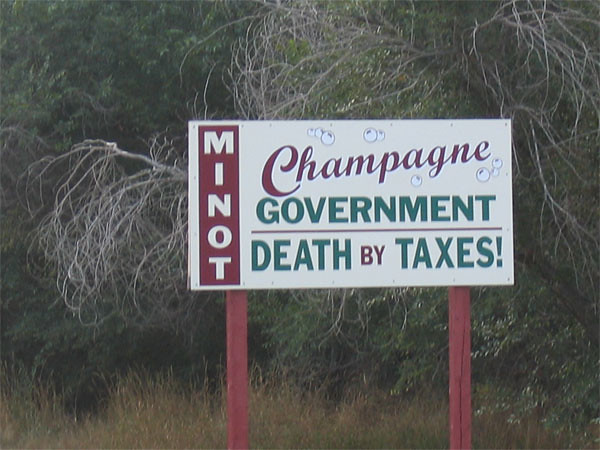A realistic photograph taken from a moving car captures a stark contrast in the landscape. In the background, a densely populated forest flourishes with well-grown trees adorned in abundant green leaves. In the foreground, several trees stand bare, their branches almost devoid of life, suggesting they might be dead. Beneath these trees, a layer of shrubbery and bushes is visible, transitioning into tall, thick grass with a blend of light green and brown hues.

At the center of the image is a distinctive sign supported by two orange wooden posts. The sign itself is completely white. Bold red cursive lettering spells out "Champagne," while below it, in green, the words "Government Death by Taxes" are prominently displayed. To the left side of the sign, a red rectangle features the word "MINOT" in white letters. The juxtaposition of vibrant forest life and the somber message on the sign creates a striking visual commentary.